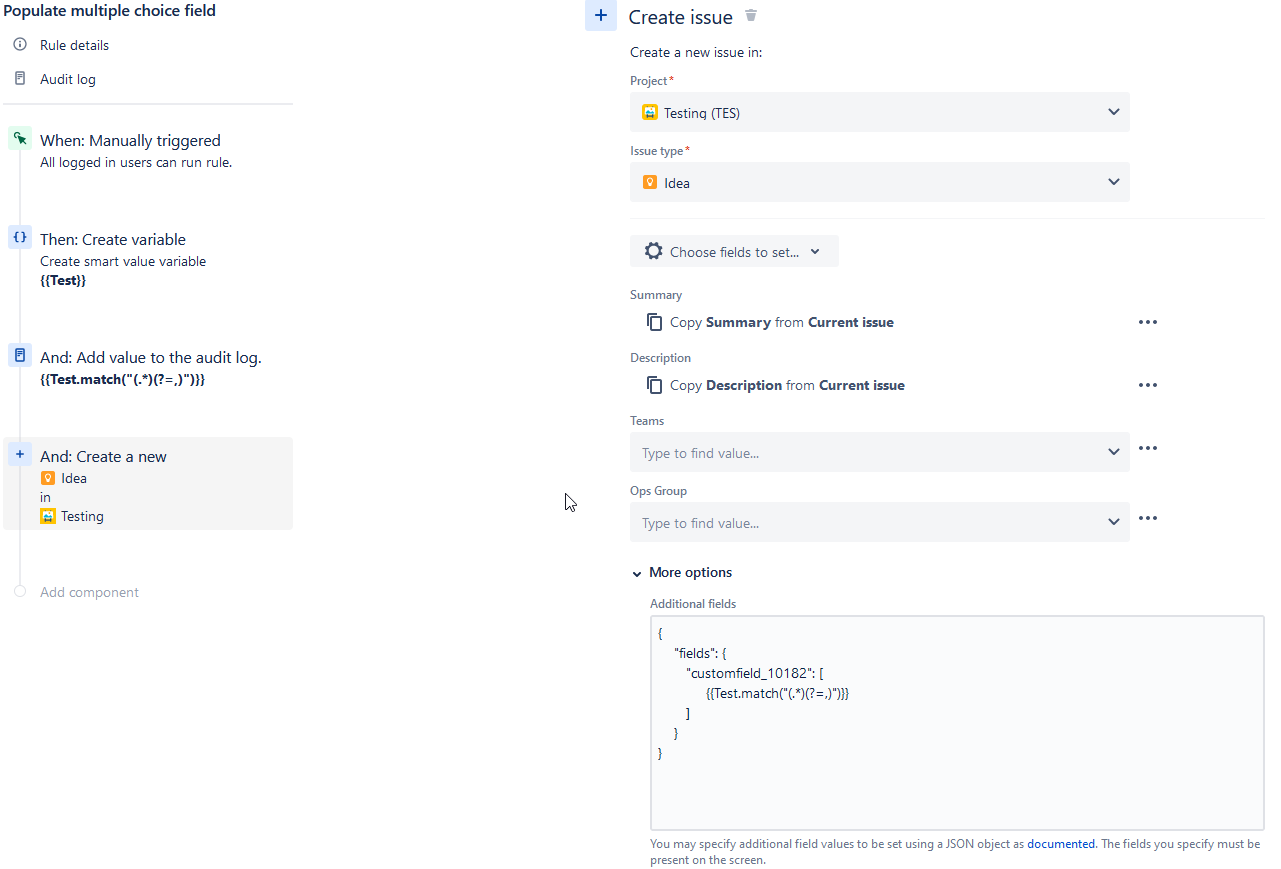The image depicts a highly detailed technical web page with a predominantly white background, designed for managing and configuring various rules and settings.

**Top Left Section:**
- The header reads "Populate Multiple Choice Field" with an icon of an eye enclosed in a circle for additional rule details.
- Directly below this, the text "Audit Log" is displayed.
- Following the "Audit Log" text, the instruction "When manually triggered all logged-in users can run rule" is noted.
- Below these instructions, there are options: "Create Variable", "Create Smart Value Variable", "Test", and "Add Value to the Audit Log".
- Additionally, it mentions "Test Match" accompanied by unspecified symbols.
- A notable feature is a plus sign with the text "Create a New Idea in Testing".

**Right Side Section:**
- The right part of the page features a plus sign labeled "Create Issue" with a trash can icon next to it.
- Another command reads "Create a New Issue in Project" followed by a red asterisk indicating a required field.
- The text "Testing T S" is displayed with a pull-down arrow for selection.
- "Issue Type" is noted with another red asterisk.
- A text box labeled "Idea" includes a pull-down arrow for additional options.
- Following this is a box with a pull-down menu labeled "Choose Fields to Set".
- Underneath, there is a section titled "Summary" with the subtext "Copy Summary from Current Issue".
- The "Description" field similarly reads "Copy Description from Current Issue".
- Further down, the text reads "Teams" with a text box labeled "Type Define Value".
- The "Ops Group" is another text box also labeled "Type Define Value".
- Below these, there are expandable options for "More Options" and "Additional Fields".
- A rectangular text box is filled with a large amount of characters and specific details such as "fields:" followed by a colon and parenthesis, and "asterisk custom field underscore" accompanied by a sequence of numbers.